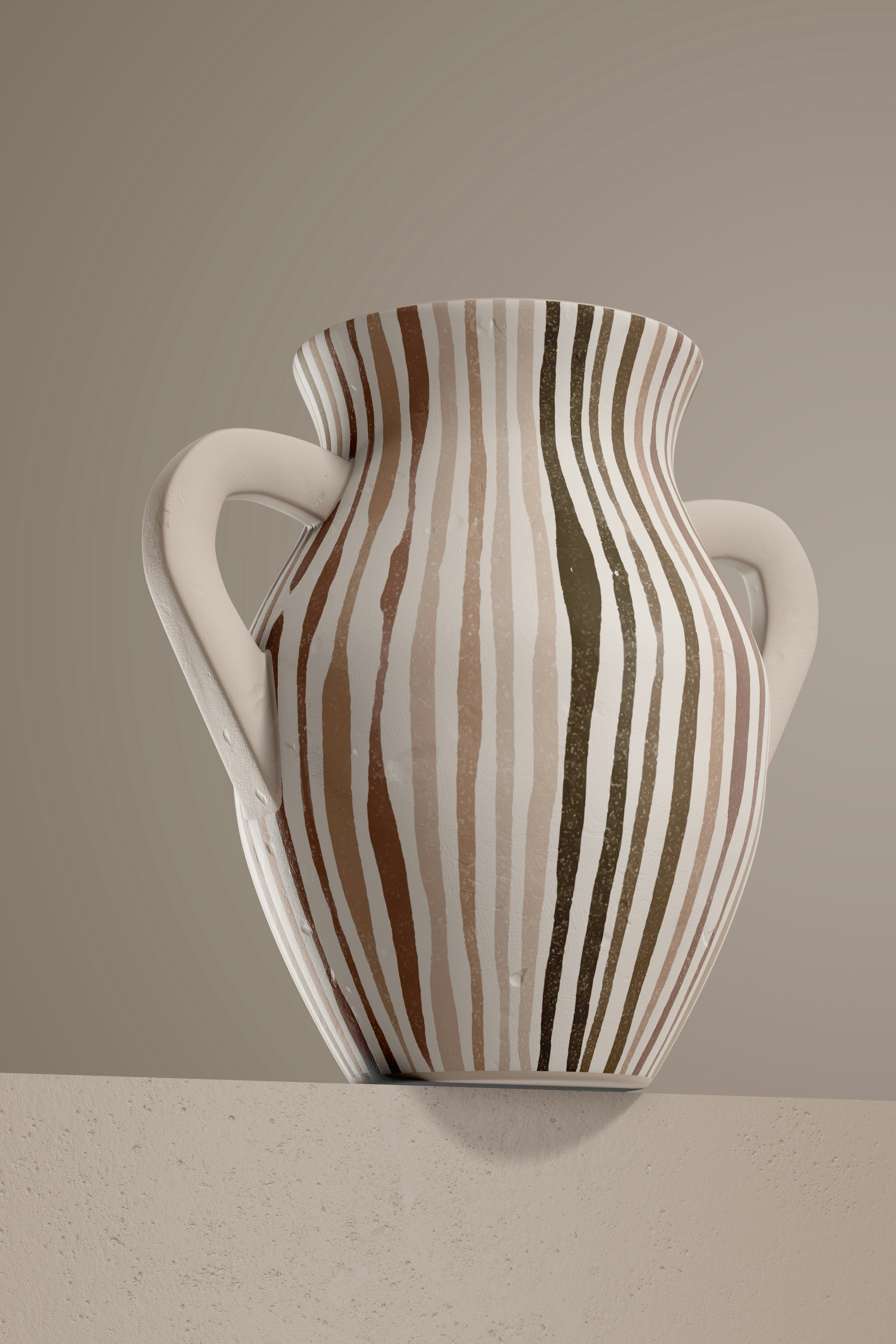The image depicts a ceramic vase with a distinctive curvy shape, featuring two unpainted, squared handles jutting out from opposite sides. The vase, made of light-colored clay, rests on a beige stone wall with a darker beige wall serving as the backdrop. It boasts hand-drawn vertical stripes in various shades—ranging from very dark brown, medium brown, and rusty red to lighter, camel sand and peachy tones—created in a freehand style, resulting in lines of varying widths. The handles resemble ears and provide a unique squared-off grip. Additionally, there are noticeable notches at the bottom of the vase, adding to its character. The overall appearance of the vase, despite its rough stripes and imperfections, makes it a particularly striking piece.